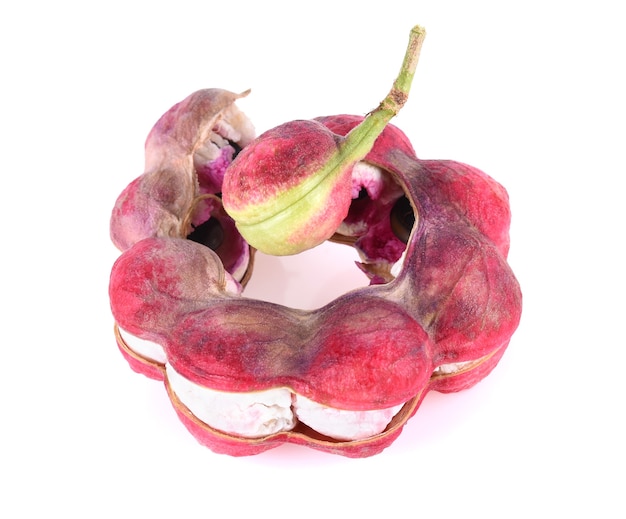In this image, we observe a peculiar and intriguing fruit that appears quite exotic and possibly tropical in nature. The centerpiece of the composition is a round, bumpy, hard-shelled fruit that is predominantly red. The red exterior seems like a protective shell that has begun to crack open, revealing white-colored inner sections. In the center, a distinctive fruit or nut is attached to a green stem; it emerges upwards and is characterized by a greenish hue with a hint of red at the top and bottom.

Surrounding the central fruit, there are several segments or pods arrayed in a circular pattern. Each pod appears to have been part of the original fruit structure, possibly indicating it has split into eight segments. These segments exhibit varied colors, including pink, lavender, and pale brown, suggesting potential decay or insect damage. Some segments have cavities, indicating that smaller pods or seeds have been removed from inside. The overall appearance gives a sense of a disassembled or partially eaten fruit, with remnants of what might have once been intact and whole. The image is set against a white background, highlighting the vivid and contrasting colors of the fruit and its components.